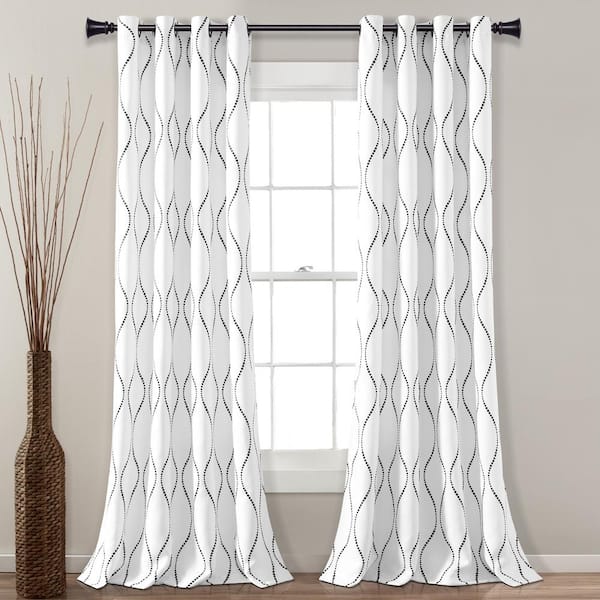This image features a tall, white-framed window flanked by partially open, symmetrical white curtains showcasing a subtle yet elegant black, wavy dotted pattern. The curtains hang from a metal curtain rod positioned at the top of the window. The room itself is bathed in neutral tones, with light gray walls and a light hardwood floor that is just barely visible in the frame. Positioned to the left of the window is a decorative wicker vase, tall and intricately braided, filled with faux sticks that rise to about one and a half feet from the floor, extending nearly to the height of the curtains. This meticulously staged setting emphasizes the delicate, flowing nature of the drapes, presenting a serene and cohesive aesthetic.